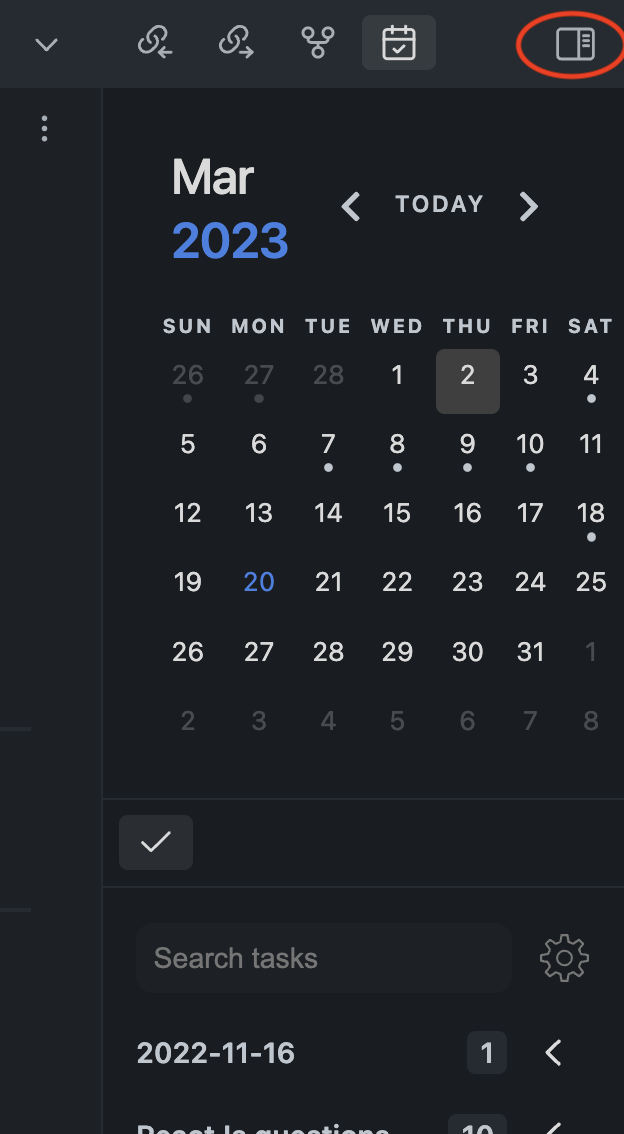This image is a detailed screen capture of a digital calendar interface. At the top, there is a toolbar with several gray icons: a down arrow, two paper clip or link icons, one with a back arrow and the other with a forward arrow. Next to these are three interconnected circles, a calendar icon, and a newspaper icon with a red-orange circle around it.

Moving down, a black side panel displays three gray dots. Adjacent to this panel, the calendar section indicates "MAR" in white text and "2023" in blue. Like the toolbar, it features back and forward arrows with "Today" marked in white-gray. The calendar view shows the days of the week from Sunday to Saturday. The last few days of the previous month (26th, 27th, and 28th) are grayed out. The date Thursday, the 2nd, is highlighted with a gray box, showing days through the 8th of the following month.

Further down, there is a gray box containing a white checkmark, followed by a search bar labeled "Search task" with a small cogwheel icon beside it. The section below shows the date "2022-11-16" accompanied by a box with the number one and an arrow. Below this, there is partially visible white text beginning with "reset," followed by a cut-off word and a box that appears to contain a number starting with '10,' but the rest is not fully visible. Beside this, a white arrow is also depicted.